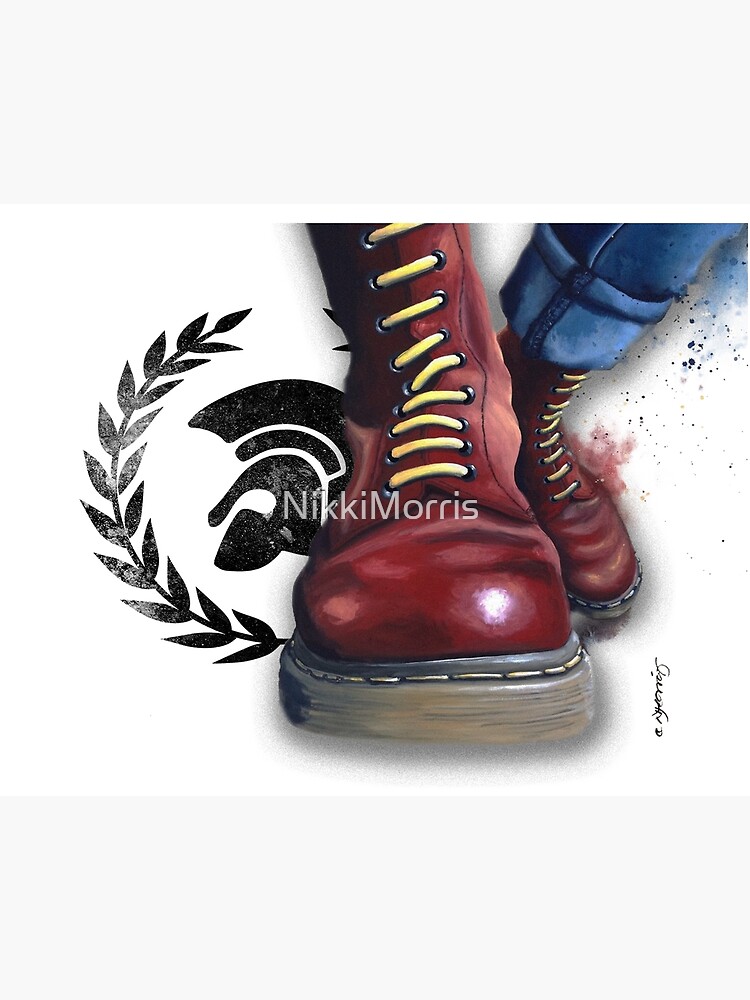This image depicts a detailed drawing of a pair of striking, maroon-colored boots resembling Doc Martens, accented with vibrant yellow laces and sturdy, light brown soles with white stitching connecting the leather upper to the sole. The right boot is prominently displayed, facing forward and shining as if reflecting light, with its heel juxtaposed against the background boot, which appears slightly lifted as though stepping. The person wearing the boots has their blue jeans cuffed just above the ankle, revealing a partial view of the leg. Across the middle of the artwork, the name "Nikki Morris" is watermarked in white, all one word, adding a possible brand identifier. The composition is framed within off-white borders at the top and bottom, featuring splatters of blue and red paint around the jeans and left boot, suggesting an artistic flair. Additionally, there is a black, abstract logo in the background depicting a Roman helmet encircled by a laurel wreath, enhancing the aesthetic appeal of this intricate and somewhat cartoonish depiction, with a barely legible vertical signature in cursive at the bottom right.